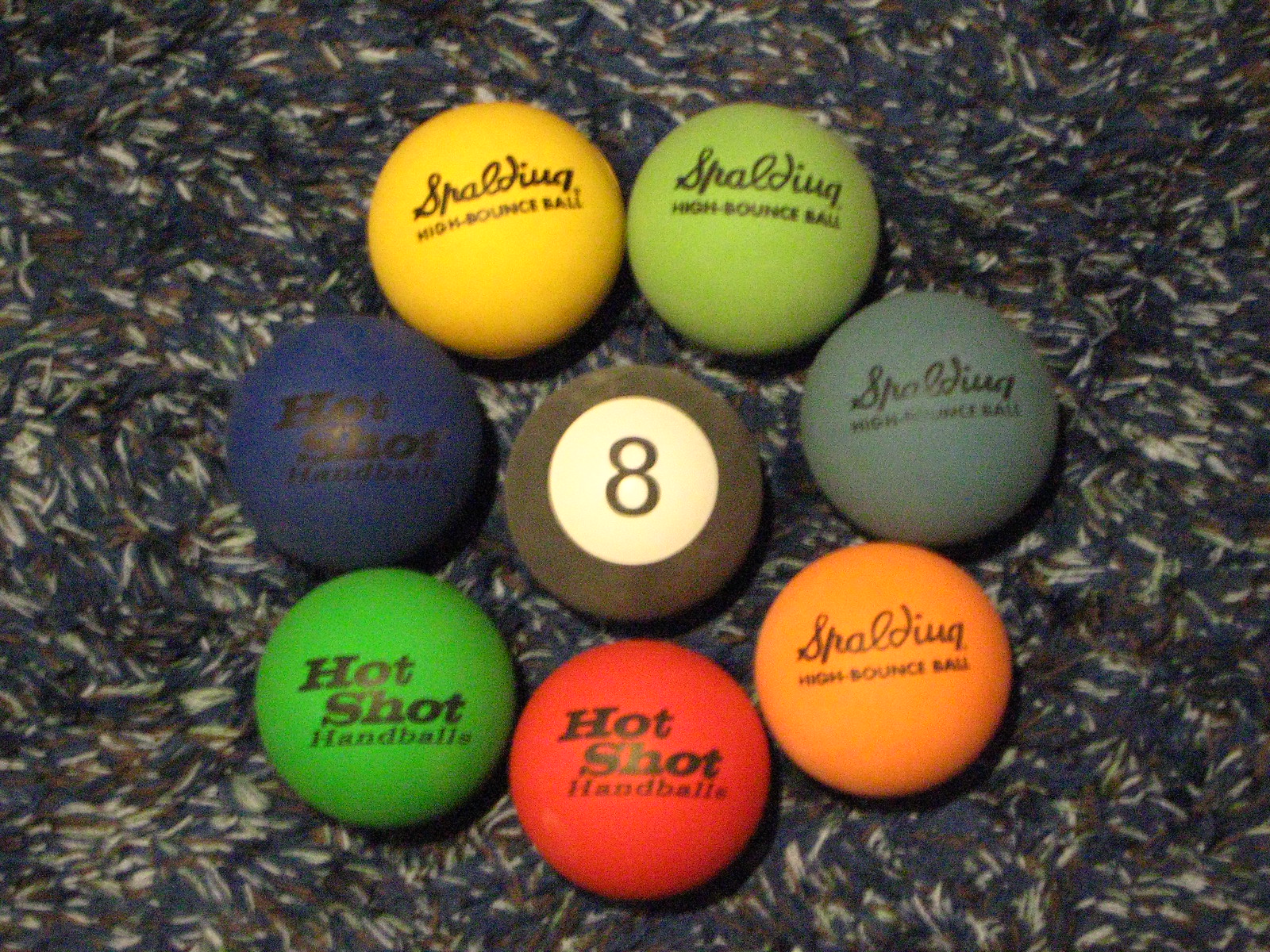In the image, we see eight hand balls of varying colors, arranged with seven forming a circle around one central ball. These balls are placed on a carpet that primarily appears dark blue with white fibers scattered throughout. The outer ring of hand balls includes a blue one, a bright green one, a reddish one, an orange one, a dark blue one, a light green one, and a yellow one. Three of these outer balls are labeled "Hot Shot Hand Balls" while the other four are marked "Spalding High Bounce Ball." The ball in the center is designed to resemble an eight ball from a pool set.